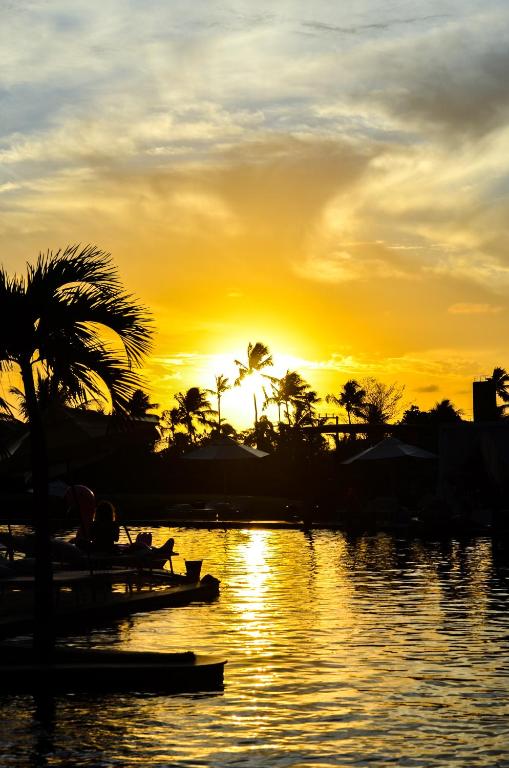The photograph captures a breathtaking sunset in a tropical setting, with a vibrant palette dominated by yellowish-orange hues around the sun, which sits near the center of the image. The sky above is a mix of blue, gray, and yellow, interspersed with beautiful clouds that partially obscure the blue sky. The vibrant colors of the sunset are beautifully reflected in the water below, possibly an ocean or river. The foreground is a vivid silhouette, featuring elements of nature and civilization: towering palm trees on the left, small pavilions, various buildings, and boats. These dark silhouettes are set against the glowing backdrop, stretching across the lower half of the image into the water, enhancing the ethereal quality of the scene. The overall composition, with its stark contrasts and rich colors, evokes a serene yet dramatic tropical evening.